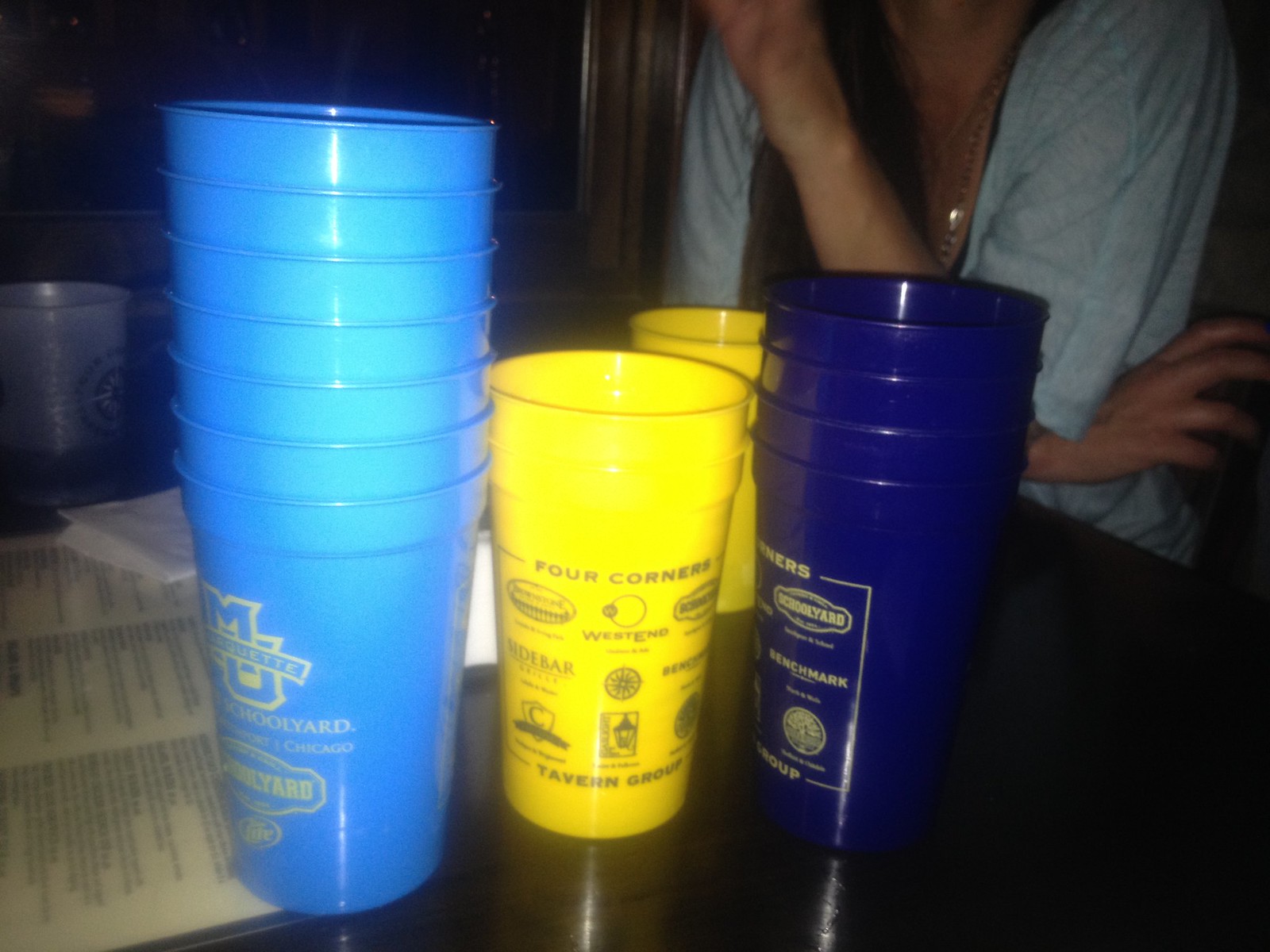The color photograph, taken inside a dimly lit restaurant or bar, captures a dark brown wooden table in the foreground. Stacked on the table are various plastic drinking cups: a stack of light blue cups on the left, standing the tallest at seven cups high, two yellow cups in the middle, and four dark navy blue cups on the right. Each cup appears to have multiple logos, with the central yellow cup distinctly featuring the text "Four Corners." To the left of the light blue cups, a laminated, three-part menu with off-white cream paper and black, unreadable text stretches towards the background. In the background on the right, partially obscured by shadow, an individual's torso is visible from the neck to the elbows, with their left hand extending out of frame. The use of flash highlights the cups and the table, while the rest of the environment remains shrouded in darkness.